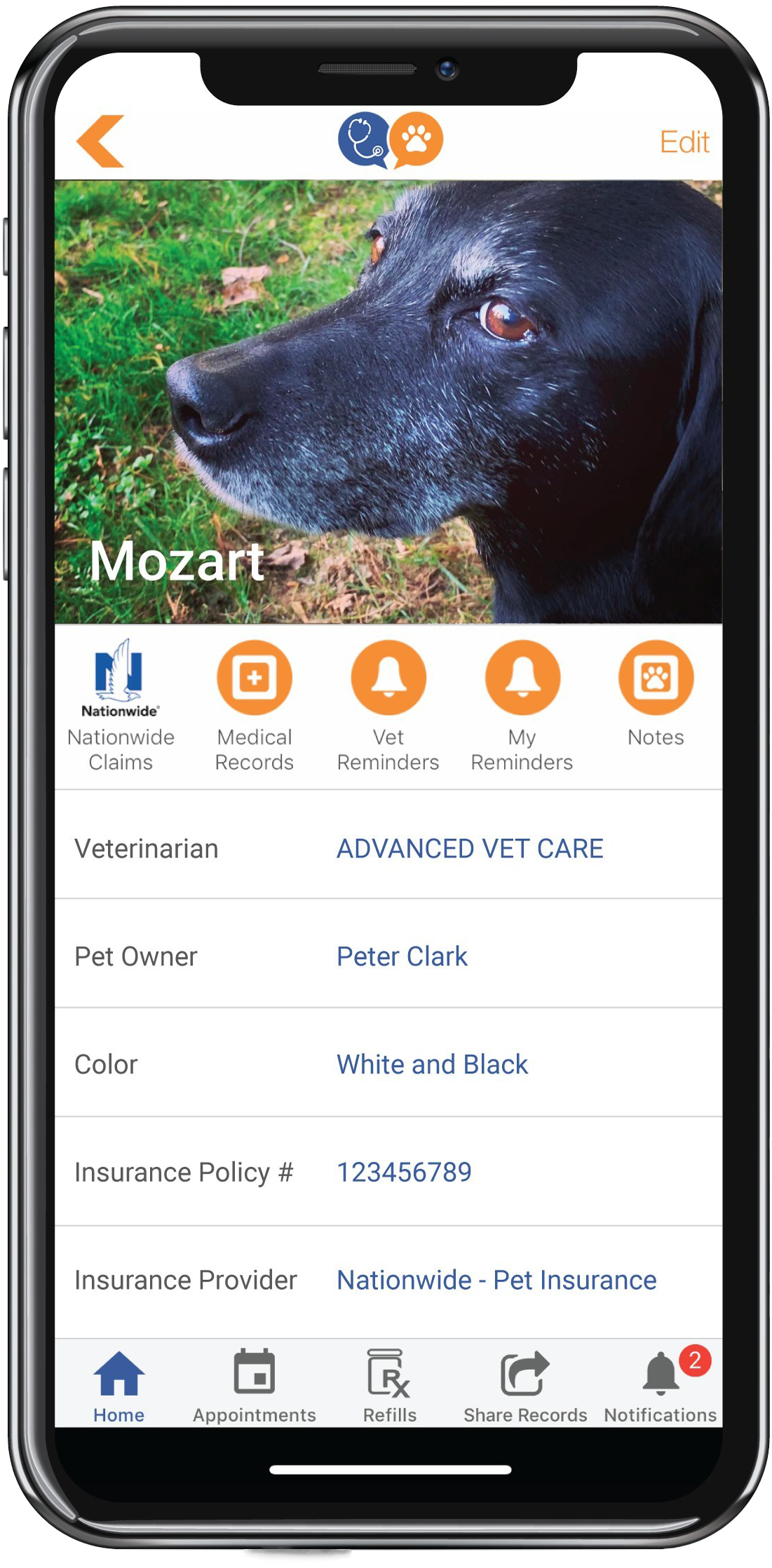The image showcases a phone screen bordered by a grayish-silver frame with a thin black inner edging. At the bottom center, there's a small white bar extending horizontally about an inch. The top features a black tab about an inch from the left, rising and ending an inch from the right, with a gray speaker line and a blue camera dot on it.

Below this, on the left side, a half-inch white border contains a bolded orange greater-than sign pointing leftwards, accompanied by a blue circle with a white stethoscope icon. Adjacent to it, an orange circle with a white dog paw is marked with the word "Edit" in orange.

Central to the screen is a three-inch close-up image of a dog's head, with black fur and brown eyes facing left, set against a grassy background. In the bottom left corner of the image, the name "Mozart" is boldly written in white.

Below the image, the Nationwide logo is on the left next to the phrase "Nationwide Claims". Four orange circles follow, each containing a white icon: a square with a plus sign, two bell icons, and a square with a dog paw imprint. Each circle is labeled respectively: "Medical Records", "Vet Reminders", "My Reminders", and "Notes". These sections are separated by thin gray lines.

Further down, the screen lists details in black text on the left: "Veterinarian", "Pet Owner", "Color", "Insurance Policy Number", and "Insurance Provider". To the right, information in blue reads: "Advanced Vet Care", "Peter Clark", "White", and a numeric sequence from 1 to 9. "Nationwide Pet Insurance" is also listed in blue.

At the bottom left corner is a blue home icon labeled "Home", followed by black text for "Appointments" with an icon, "Refills" with an icon, "Share Records" with an icon, and "Notifications" with a bell icon. A red circle with a white number "2" is positioned to the right of the notification bell.